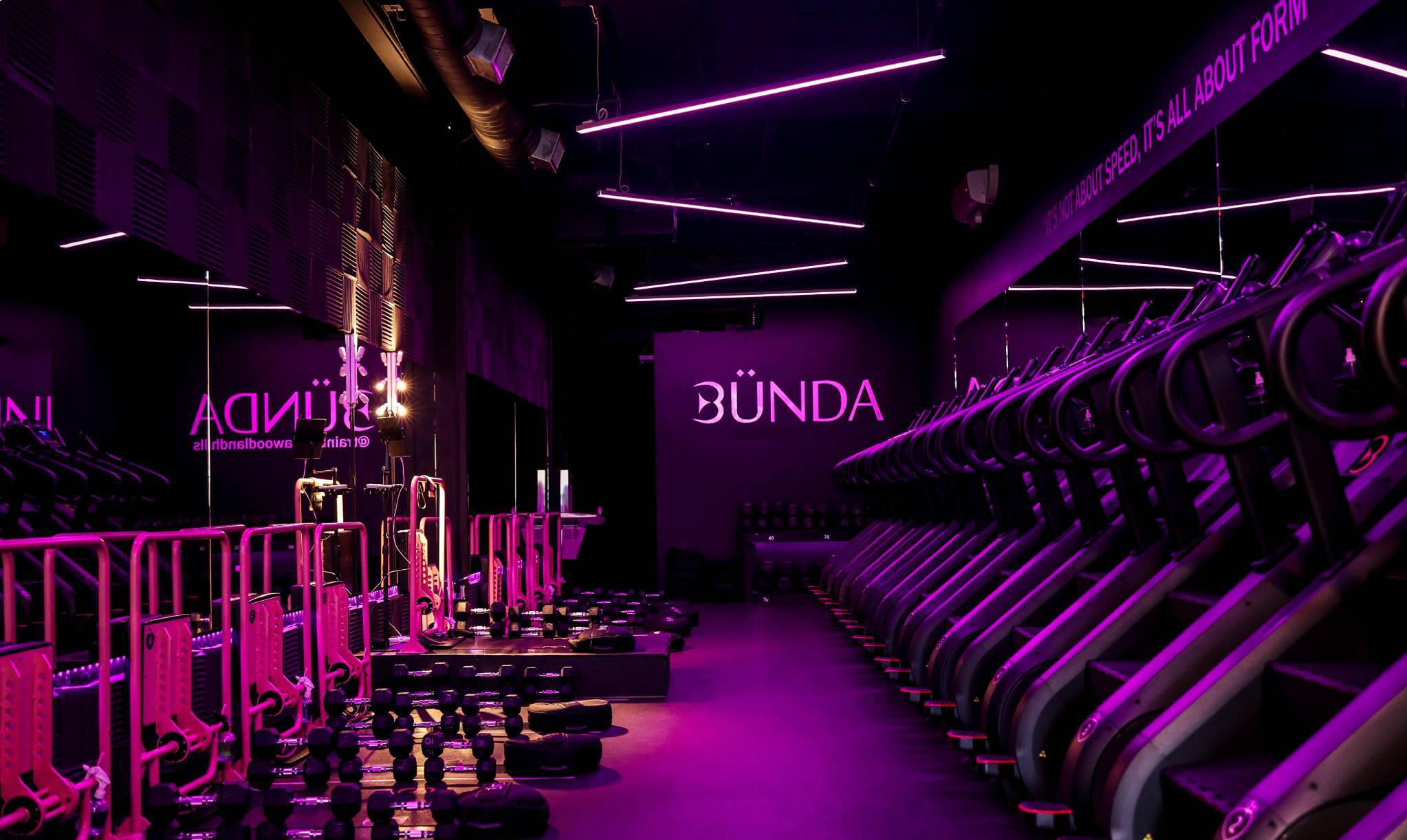This photograph captures the interior of a dimly lit, empty gym, casting a magenta or purplish hue across the entire space. The focal point is a back wall illuminated with a glowing sign that reads "Bunda," likely the name of the fitness center or studio. The gym is arranged with various equipment: on the right side, several electronic stair climber machines are lined up against the wall; on the left side, there is a neatly organized array of black barbells and hand weights. A closely placed row of mirrors reflects the gym equipment, adding depth to the view. The overall setting suggests a focus on proper form over speed, reinforced by a sign that, presumably, states "It’s not about speed, it's all about form." This combination of sleek, modern equipment, strategic lighting, and thoughtful layout contributes to an inviting, professional atmosphere intended for disciplined workout sessions.